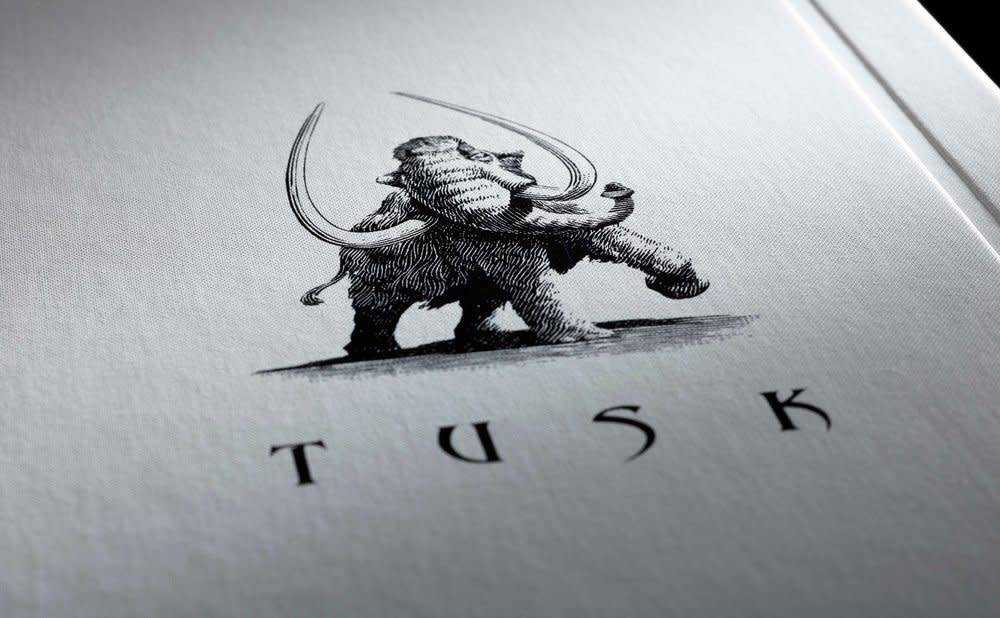The image appears to be a book cover with a white, hardcover design. Dominating the center of the cover is a finely detailed, black-and-white sketch of a woolly mammoth. The mammoth is depicted with its body primarily facing to the right, while its head is turned toward the viewer, showcasing intricate details like its fur and textured trunk. The trunk is adorned with notches and swings up and to the right, and the mammoth's long, curved tusks, which point toward each other, add to its imposing presence. The artist has skillfully used a combination of black ink and white space to highlight different parts of the mammoth, giving it a textured, almost three-dimensional appearance. The fur is intricately drawn, with some areas appearing darker due to shadowing. Below the image of the mammoth, the word "TUSK" is displayed in capitalized, sharp-edged letters, creating an impression of simplicity and elegance. The overall image of the mammoth appears to be walking on its shadow, which is also thoughtfully rendered in fine lines. An embossed line running through the cover suggests the seam where the book would open. The entire layout, along with the mammoth’s powerful depiction, suggests a narrative with a historical or fantasy element.